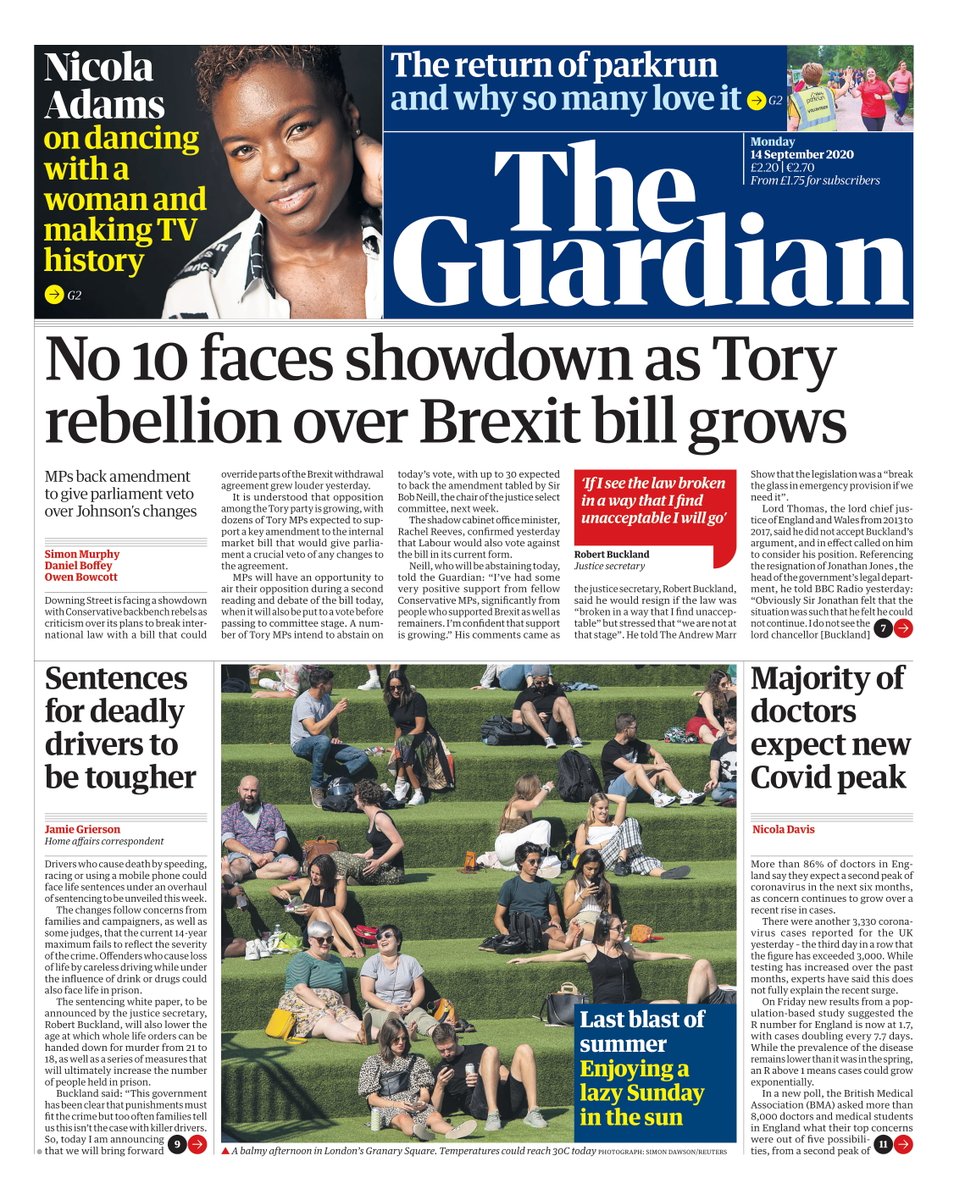Front Page of The Guardian: A Detailed Breakdown

**Top Section:**
- **Small Square Box (Black Background):**
  - Features a close-up picture of a person (presumably Nicola Adams) with short black hair and a slight smile. The individual is wearing a white shirt with black designs. Their left hand is resting on the back of their neck.
  - Caption: "Nicola Adams on Dancing with a Woman and Making TV History."

- **Rectangular Box (Blue Background):**
  - Title: "The Guardian" in large white bold print.
  - Subheading: "The Return of Park Run and Why So Many Love It."
  - Small inset picture of people high-fiving during a race.

**Middle Section:**
- **Headline:** "No Tan Faces Showdown As Tory Rebellion Over Brexit Bill Grows" in bold black print.
- **Article Summary:**
  - "MPs Back Amendment To Give Parliament Veto Over Johnson's Changes."
  - Written by Simon Murphy, Daniel Boffey, and Owen Bokud (names in red).
- **Additional Navigation:**
  - Black circle with the number 7 and a red circle with a white right-pointing arrow, suggesting the option to read more of the article.

**Bottom Section:**
- **Large Picture:**
  - Scene of people sitting on grassy steps or steps with artificial grass in London's Granary Square on a warm afternoon.
  - Caption: "A balmy afternoon in London's Granary Square. Temperatures could reach 30 degrees Celsius today."
  - Photo credit: Simon Dawson of Reuters.
  - Observations: Most people are wearing short-sleeved shirts and shorts, with a few in long pants and one in a skirt. The crowd is predominantly white, with one young lady who appears to have a dark tan or light-skinned black complexion.
  - Inset caption: "Last blast of summer, enjoying a lazy Sunday in the sun."

**Side Articles:**
- **Left Side:**
  - Title: "Sentences for deadly drivers to be tougher" by Jamie Gerson.
  - Additional content indicated with an arrow to read more.

- **Right Side:**
  - Title: "Majority of doctors expect new COVID peak" by Nicola Davis.
  - Additional content indicated with an arrow to read more.

This thorough descriptive caption encapsulates the contents and layout of the front page of an issue of The Guardian, covering key headlines, visual elements, and article snippets.